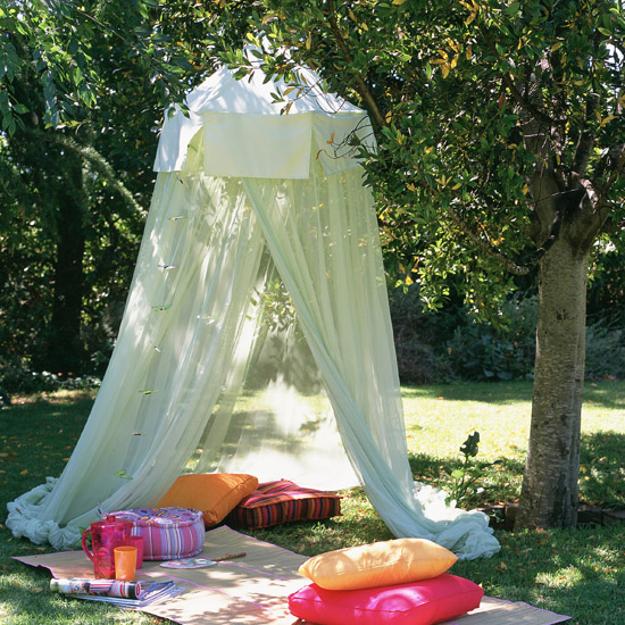A picturesque summer day unfolds in a verdant park with towering, full-bloom trees casting a serene canopy of vibrant green leaves. The sunlight filters gently through the leaves, illuminating a delicate, gauzy white tent draped elegantly from the robust branches, creating a cozy, shaded nook. This ethereal tent, shimmering as sunlight dances through it, pools gracefully onto a soft beige blanket spread out on the lush grass below. Inside this inviting setup rests an array of colorful pillows in oranges, pinks, reds, and blues, artfully arranged to offer comfort. A small pink and orange striped cushion and a smaller blue and pink cushion add to the vibrant tapestry of colors. 

On the blanket, amongst the cushions, lies a picnic scene: an inviting pink acrylic pitcher, likely filled with cooling ice, and two matching glasses in orange and pink hues. Nearby, a few magazines suggest someone has been leisurely reading. The entire setting, with the fluttering white tent and its splash of lively colors, exudes a romantic and enchanting ambiance, perfect for a charming picnic or an intimate outdoor date amidst nature’s splendor.